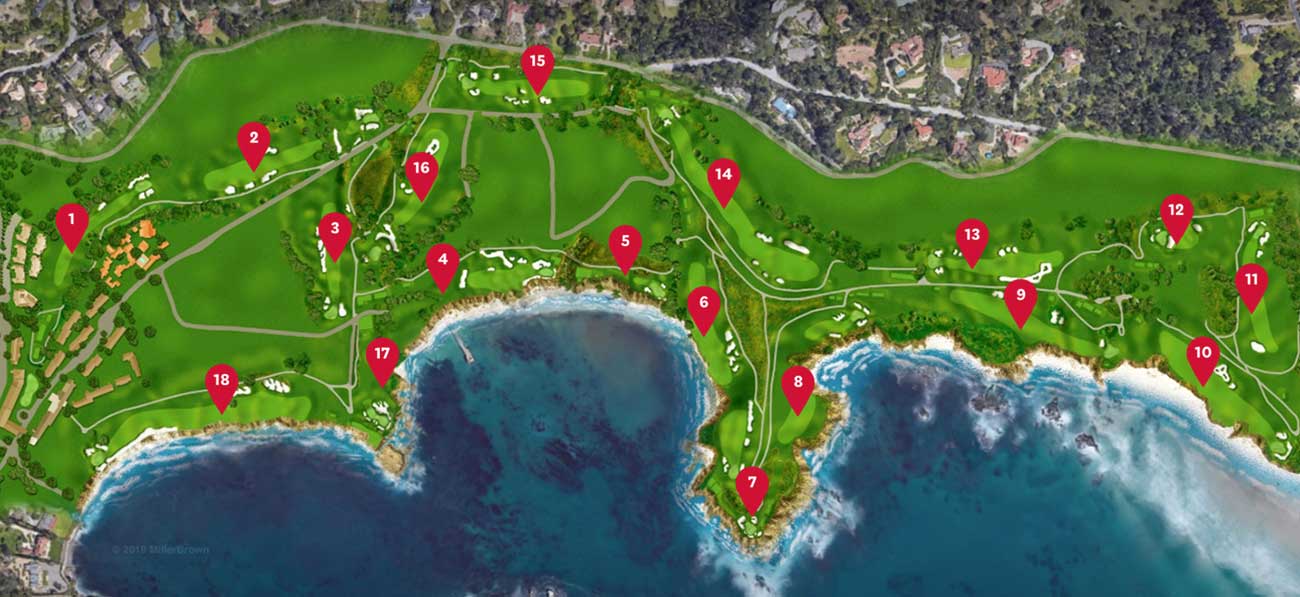The image is an aerial view of what seems to be a highly detailed graphical map of a coastal neighborhood or possibly a golf course nestled within a vibrant, green forested area. The region includes a striking rocky coastline with large waves, especially prominent on the right side of the image. The map showcases two small peninsulas and various inlets along the shoreline.

Central to the image is a section that features well-defined fairways, trails, tree lines, and sand traps typical of a golf course. This area is overlaid with little red geomarker tags, rounded on the top and pointy at the bottom, each displaying white numbers from 1 to 18, possibly marking holes or plot locations. Roads and small buildings are visible, suggesting development is underway.

To the left of the central peninsula lies a gulf of water and additional outcroppings of land, as well as a small city area in the bottom left corner transitioning to farmland. The bottom right of the image reveals clouds or the foam from crashing waves, adding to the dynamic coastal scenery.